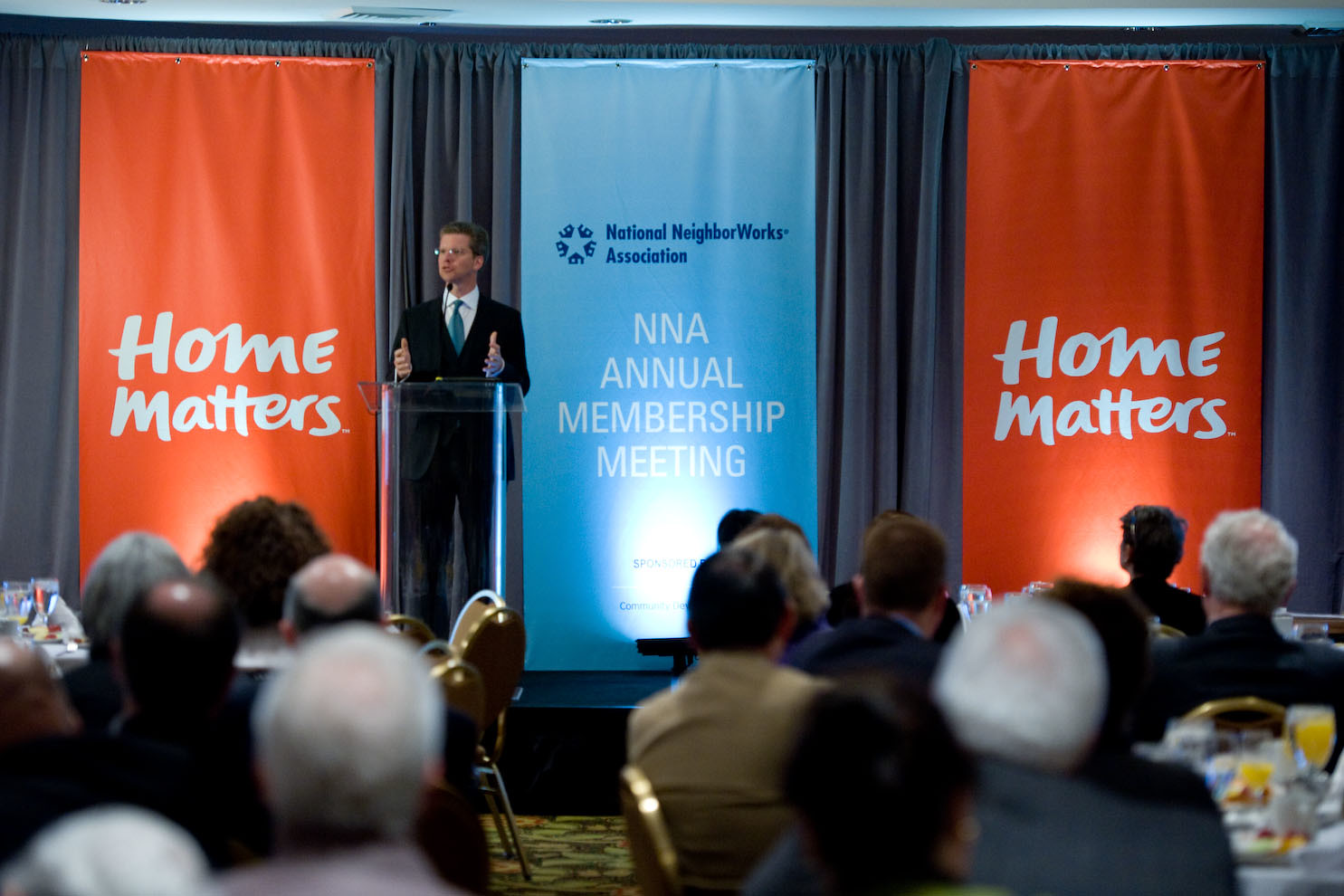In a well-lit presentation room, a man stands on a stage at a clear plastic lectern, addressing an audience. He is dressed in a black suit paired with a white shirt and a blue tie, and he wears glasses. His short brown hair is neatly groomed as he gestures with both hands, speaking into a microphone and looking towards his left. The backdrop features a navy blue curtain with three prominent banners: the two outer banners are orange and display the phrase "Home Matters" in elegant white cursive, while the central blue banner reads "National Neighbor Works Association, NNA Annual Membership Meeting."

In the foreground, the backs of the audience members are visible, slightly blurred. They are seated at tables adorned with various drinks, including glasses of orange juice, along with plates of food. The crowd, comprised largely of elderly individuals, attentively listens to the speaker. The room's ambiance is highlighted by a brown and green patterned carpet, adding to the detailed setting of this National Neighbor Works Association event.